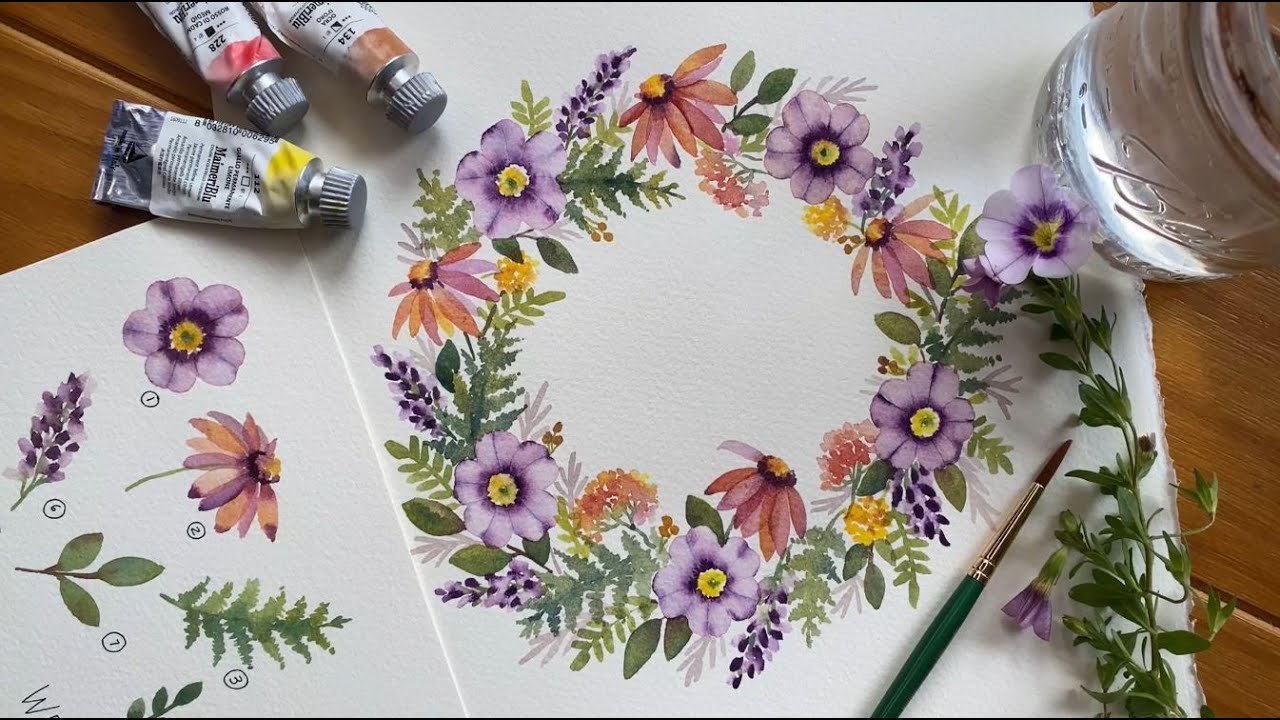This image captures a detailed artistic workspace centered around a floral-themed painting. Dominating the composition is a circular wreath painted on a piece of white paper, featuring a harmonious blend of purple, pink, red, and yellow flowers interspersed with lush green leaves. Adjacent to this main artwork, there is a separate sheet displaying watercolor sketches, each illustrating distinct phases and types of the flowers and leaves found in the wreath. These sketches, arrayed from left to right, depict flowers ranging from fully bloomed to wilting, accompanied by various leaf patterns.

In the upper left corner of the image, three used acrylic paint tubes are positioned against a wooden surface, each marked with a colored outline near the cap—yellow, red, and brown—indicating the respective paint colors. On the right side of the paper lies a mason jar filled with water, likely for rinsing the brushes. A paintbrush rests next to the jar, distinguished by its brass neck, green handle, and brown-tipped bristles. Between these tools, a real flower with pink petals, a purple interior, a yellow center, and cascading green leaves adds a natural touch to the artistic setup. Altogether, this detailed scene not only showcases the completed wreath painting but also provides a glimpse into the creative process and materials used by the artist.